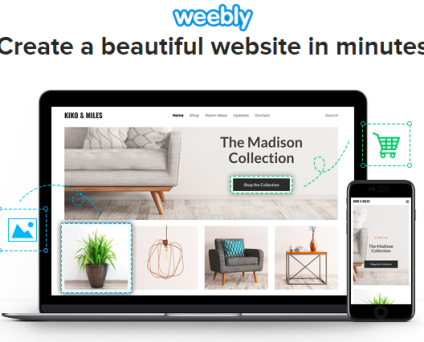A clean and detailed caption for the image described:

---

This advertisement promotes Weebly, an online platform designed for swift and easy website creation. The Weebly logo is displayed prominently in blue outline text with a white center. The tagline, "Create a beautiful website in minutes," underscores the user-friendliness of the service. Pictured are a laptop and a smartphone, both showing the same website interface, highlighting the platform's responsive design capabilities for both mobile and desktop devices.

At the top center of the advertisement, a green shopping cart icon within a green, dotted outline box draws attention, accompanied by a squiggly arrow pointing towards an interactive web design option. The middle left side features a blue squiggly line around a placeholder image area, indicating where users can upload their own visuals.

The example website on display appears to represent a furniture retailer named Kiko and Miles. This demo site includes various user interface elements such as top navigation categories, a search button, and a promotional section titled "The Madison Collection" with a prompt to "Browse the collection." The centerpiece is a modern gray couch with brown legs set against a complementary floor and background. Surrounding it are additional product images: a green plant in a brown pot, a striking red chandelier resembling an exploded whisk, a gray chair adorned with a bright blue patterned pillow, and a contemporary orange-topped end table with squared metal legs.

This advertisement effectively showcases Weebly’s versatile and sleek design capabilities tailored for e-commerce and home furnishing businesses.